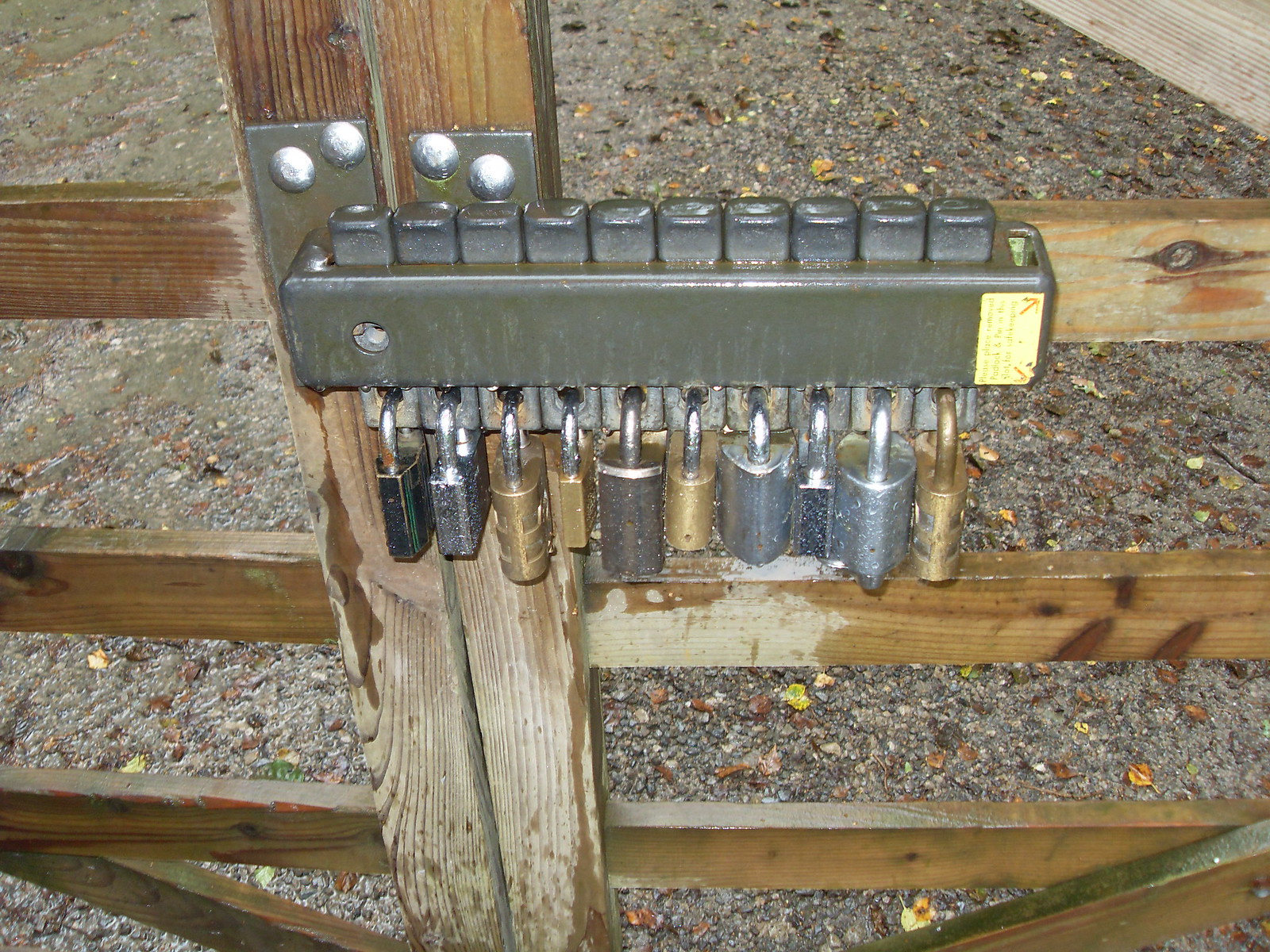The photograph depicts a wooden fence or gate with a natural light brown appearance, accentuated by visible knots and a textured grain. Central to the image are two vertical wooden posts, each adorned with bolted steel fixtures. The main feature is a large silver locking mechanism attached to the gate, with approximately ten varying padlocks hanging from it in a row. These padlocks differ in size and color, including black, silver, gold, and brown, with some exhibiting age and patina. The bottom of the image reveals a gravel or dirt ground, sprinkled with small yellow-brown leaves and patches of short light green grass. The scene suggests a robust security measure, with an interesting interplay of aged and new padlocks contributing to the fence’s fortified appearance.